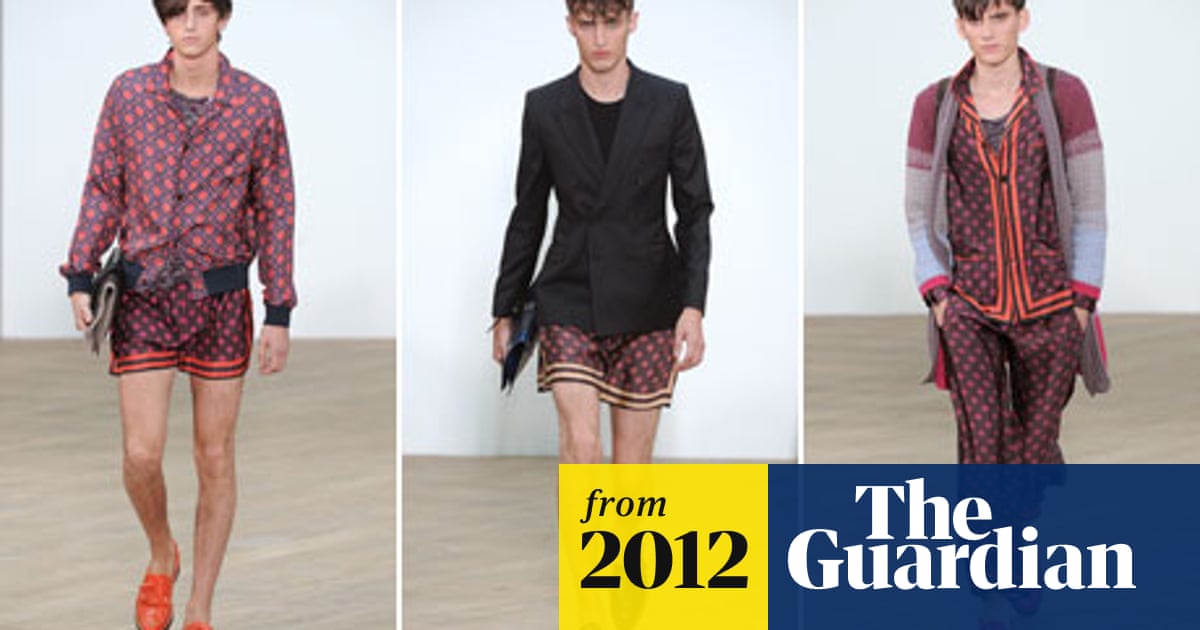The image showcases a triptych of photos featuring male models striding down a runway against a stark white backdrop and a light gray wood-toned floor. The left photo presents a model in a vibrant, busy printed bomber jacket with a dark background and red patterns. He pairs this with matching silk shorts and striking bright orange loafers. The middle image displays another model clad in a refined black blazer over the same distinctive printed shorts. Finally, the right photograph shows a model wearing a button-up shirt and long pants in the same print, complemented by a gray and burgundy cardigan. Notable textual elements include a yellow background with "from 2012" in black lettering and "The Guardian" in white text on a blue background, positioned towards the bottom right of the images.